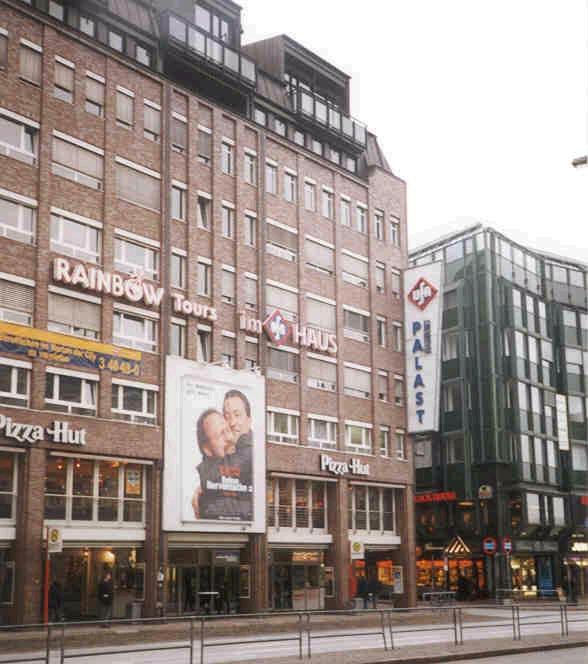The photograph captures a bustling urban scene featuring two prominent buildings. The dominant structure on the left is a red brick edifice, rising six to seven stories high, adorned with numerous windows on its facade. Notable signage on this building includes "Rainbow Tours I M H A U S" in the middle and "Pizza Hut" displayed prominently to both sides of the entrance. An eye-catching movie poster depicting two men hugging spans two to three stories on the lower section of this building. Adjacent to this brick building, on the right, stands a contemporary glass structure of similar height, housing what appears to be retail shops on the ground level. A distinctive vertical sign with blue lettering spelling "Palast" is visible on the glass building. The photograph is taken from across the street, with a metal fence visible in the foreground, indicating a bustling city setting likely outside a foreign city.